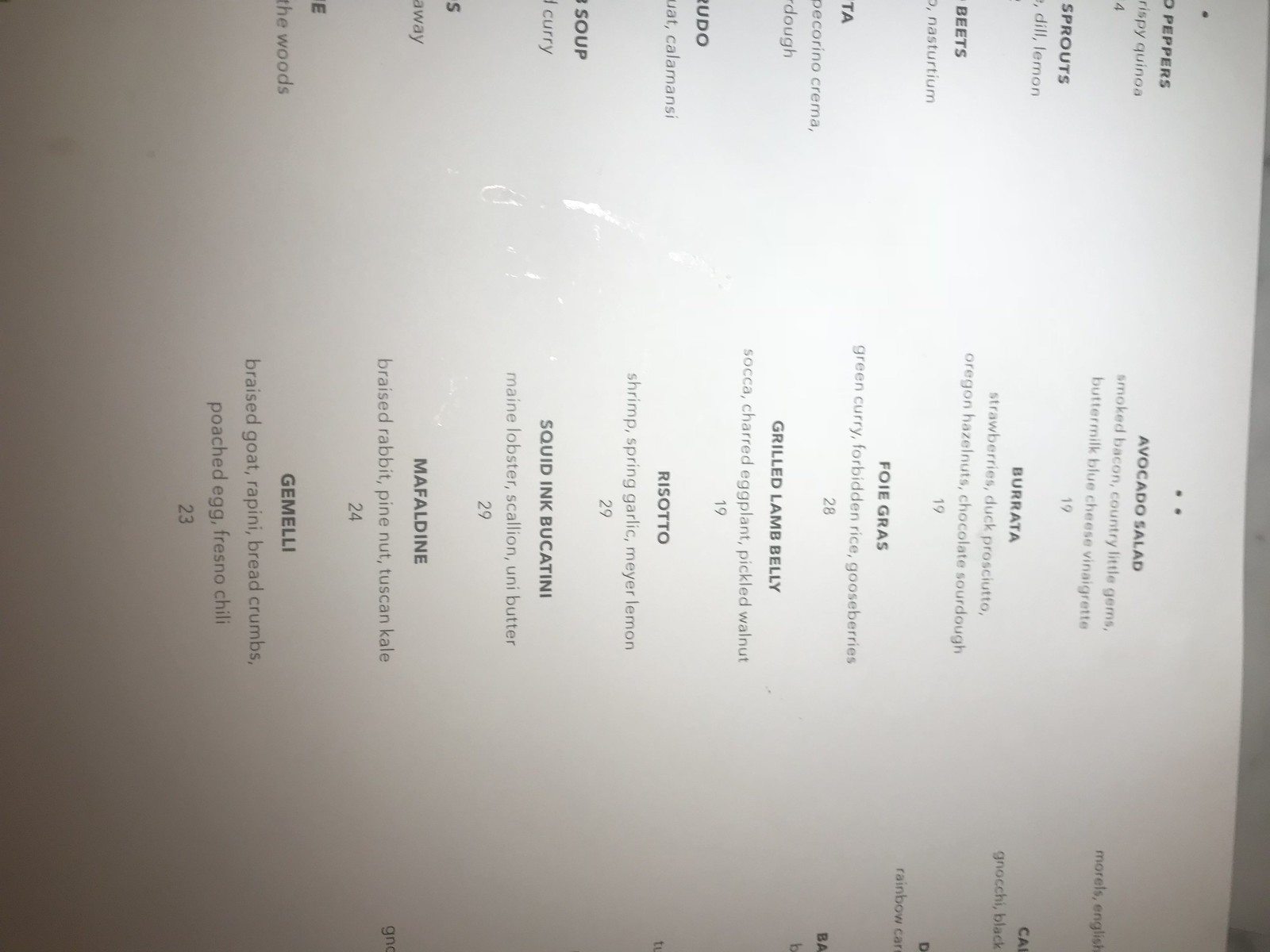Here's the polished and detailed caption:

---

This image captures a section of a sideways-oriented menu. The text is aligned with the letters facing to the right, meaning the top of the letters is directed toward the right edge and the bottom toward the left, creating columns that read from top to bottom.

At the very top of the menu, approximately one inch from the right edge, there's a snippet of text across five sections. Toward the bottom, again about an inch from the right edge, there are four sections showing brown lettering creeping in.

In the center-right of the menu, there are two dots, and directly beneath them, in large bold letters, reads "AVOCADO SALAD." Underneath this title, the ingredients for the avocado salad are listed, followed by the price "19."

Proceeding downward in large black letters:

- "BURRATA" is prominent, followed by a detailed list of ingredients in smaller, lighter text, and the price "19."
- "FOIE GRAS" is bold and black, with ingredients listed underneath and priced at "28."
- "GRILLED LAMB BELLY" is displayed, with its ingredients detailed below and priced at "19."
- "RISOTTO" is presented in bold, moving from right to left, followed by its ingredients and priced at "29."
- "SQUID INK BUCANTI" follows, with ingredients listed underneath and the price "29."
- "MAFALDINE" is next, with the ingredients beneath and priced at "24."
- Lastly, almost reaching the left side, the word "GEMELLI" is in black, followed by the ingredients in smaller text and a price of "23."

This detailed menu excerpt provides a glimpse into the offerings of an upscale dining establishment, with each dish meticulously labeled and priced.